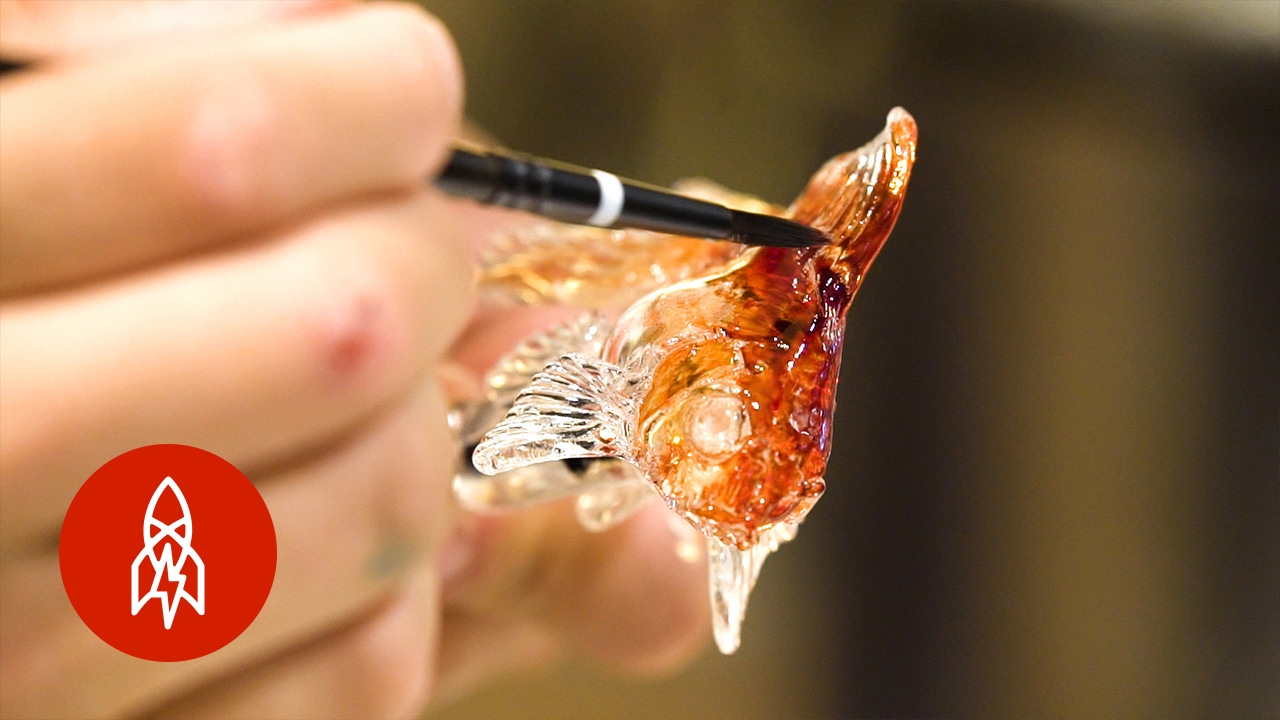The image captures a close-up view of an artist meticulously painting a glass sculpture of a goldfish. The artist, whose hand is on the left side of the image, is likely Caucasian and is using a long black brush with a white strip in the middle and an all-black tip. The hand only shows the knuckles of the first four fingers, which are slightly out of focus, while the main focus is on the glass fish. The fish, made of clear glass, has transparent white fins and is being painted with a special clear paint in a vibrant orange color that glistens while maintaining its transparency. The background is completely blurred out, drawing attention solely to the detailed painting process. In the lower left-hand corner of the image, there's a red circle featuring a white outline of a rocket with an electrical bolt running through its center. This element adds a unique touch to the overall composition of the image.